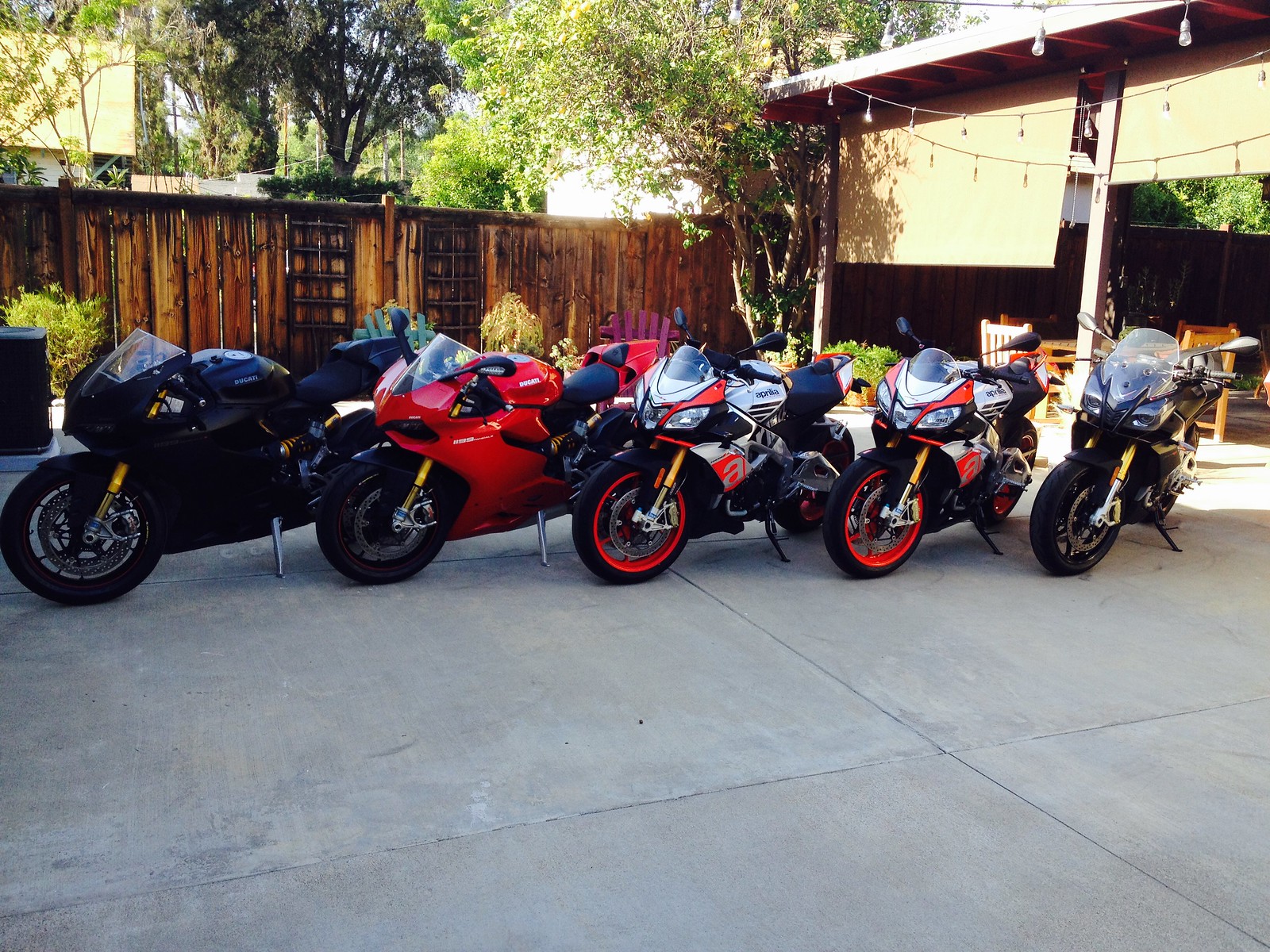The image depicts a row of five sports motorcycles parked in a courtyard with a concrete ground floor. In the background, there is a dark brown wooden fence, and to the right, a shaded dining area with tables and seating is visible, featuring a string of lightbulbs overhead. Each motorcycle is propped up by a kickstand and parked at an angle from right to left. The bike on the far left is entirely black, followed by a red motorcycle with a black seat. The third and fourth motorcycles sport a mix of silver, red, and black with black wheels that have a red trim around the rims. The last motorcycle on the right is all black and positioned almost straight ahead. The scene also includes some ladders leaning against the fence.